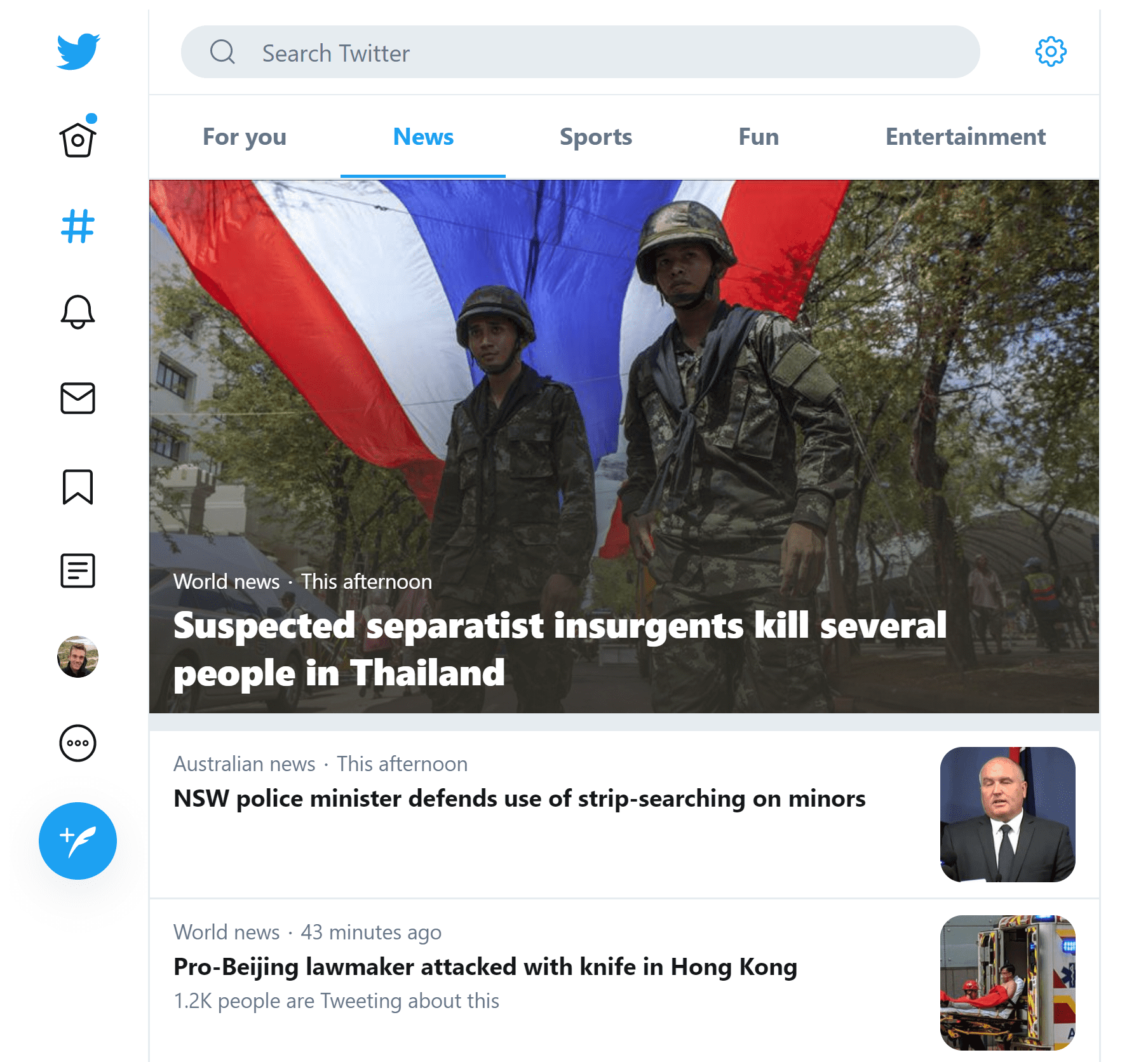The image is a vertical screenshot from the Twitter app, viewed on a webpage, smart device, or through the app interface. The background is predominantly white, reminiscent of a computer screen. On the left-hand side, there's the recognizable blue Twitter bird icon followed by several standard icons in sequence: home, hashtag (trending), bell (notifications), email (messages), bookmark, a box with lines (lists), profile picture, an option for more, a plus sign, and a blue feather for composing a tweet.

At the top, a gray bar features a magnifying glass icon adjacent to the "Search Twitter" input field, useful for conducting searches. On the far right side of the screen, there's a settings icon. Below the search bar, various tabs are visible: “For You,” “News” (currently selected and highlighted in blue and underlined), “Sports,” “Fun,” and “Entertainment.”

The central part of the image showcases a photo depicting soldiers beneath a flag or canopy with trees and other people in the background. The caption reads: "World News this Afternoon: Suspected separatist insurgents kill several people in Thailand." Below this segment, in another white background section, the caption reads: "Australia News this Afternoon: NSW police minister defends use of strip searching on minors," accompanied by a small image of the police minister.

Further down, another headline appears: "World News 43 minutes ago: Pro-Beijing lawmaker attacked with knife in Hong Kong," noting that 1.2 thousand people are tweeting about it, and includes a related picture.